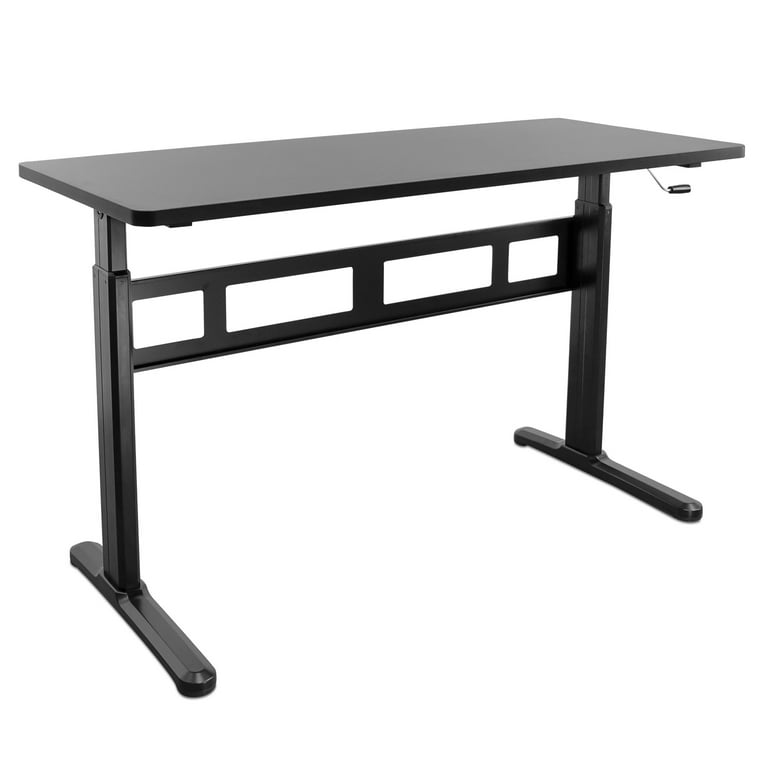The image features a realistic, black computer desk or work desk positioned against a stark white background, creating a floating effect with no shadows or other elements in view. The desk has a long, horizontal rectangular top, likely made from black wood, and is supported by a black metal frame. The legs of the desk are composed of rectangular pole frames, each with a ladder-like structure near the top that includes three horizontal rungs connecting the front and back poles. The bottom of the desk’s legs is stabilized by two rectangular strips of metal where the legs are anchored. On the right side, under the tabletop, there's a silver handle with a black circular end, suggesting that the desk might be adjustable for height. This desk appears sleek and modern, with a design suitable for a professional office environment.